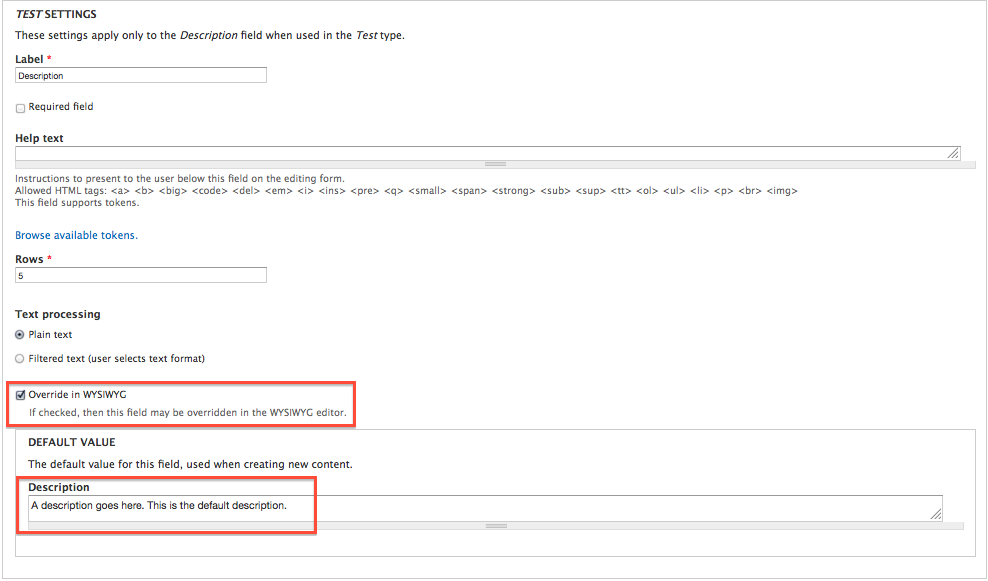**Caption:**

The image showcases a settings interface, which appears to be on either a laptop or desktop screen, specifically for configuring "Test Settings." At the top of the interface, "TEST SETTINGS" is prominently displayed in black, all-caps text, with the word "test" italicized. Below this header, it states, "These settings apply only to the description field when used in the test type."

The subsequent section has a label field marked with a red asterisk (*), indicating that it is mandatory. You can input a description in this label box. Beneath the label field is an option to mark the "Required Field," which is currently unchecked.

Further down, there's a "Help Text" field, a long space where additional information can be typed. It includes instructions for what will be presented to the user below this field on the editing form, mentioning the allowed HTML tags along with a note that this field supports tokens. A link labeled "Browse Available Tokens" in blue is provided for reference.

The next section includes a "Rows" field, also marked with a red asterisk (*), and in this example, the number "5" is specified. Following this is a "Text Processing" field where "Plain Text" is selected by default. Users also have the option to select "Filter Text" or let users choose the text format, though these options are not selected in this instance.

Further down is a checkbox for "Override in WYSIWYG," which, if checked, allows the field to be overridden in the WYSIWYG editor. This option is highlighted with a red box.

At the bottom of the interface, there's a "Default Value" section indicating the default text that appears in this field when creating new content. The default description provided is "A description goes here. This is the default description," and this section is also highlighted with a red box.

The interface is detailed and meticulously organized, clearly delineating each field and option available for the user to configure the test settings.